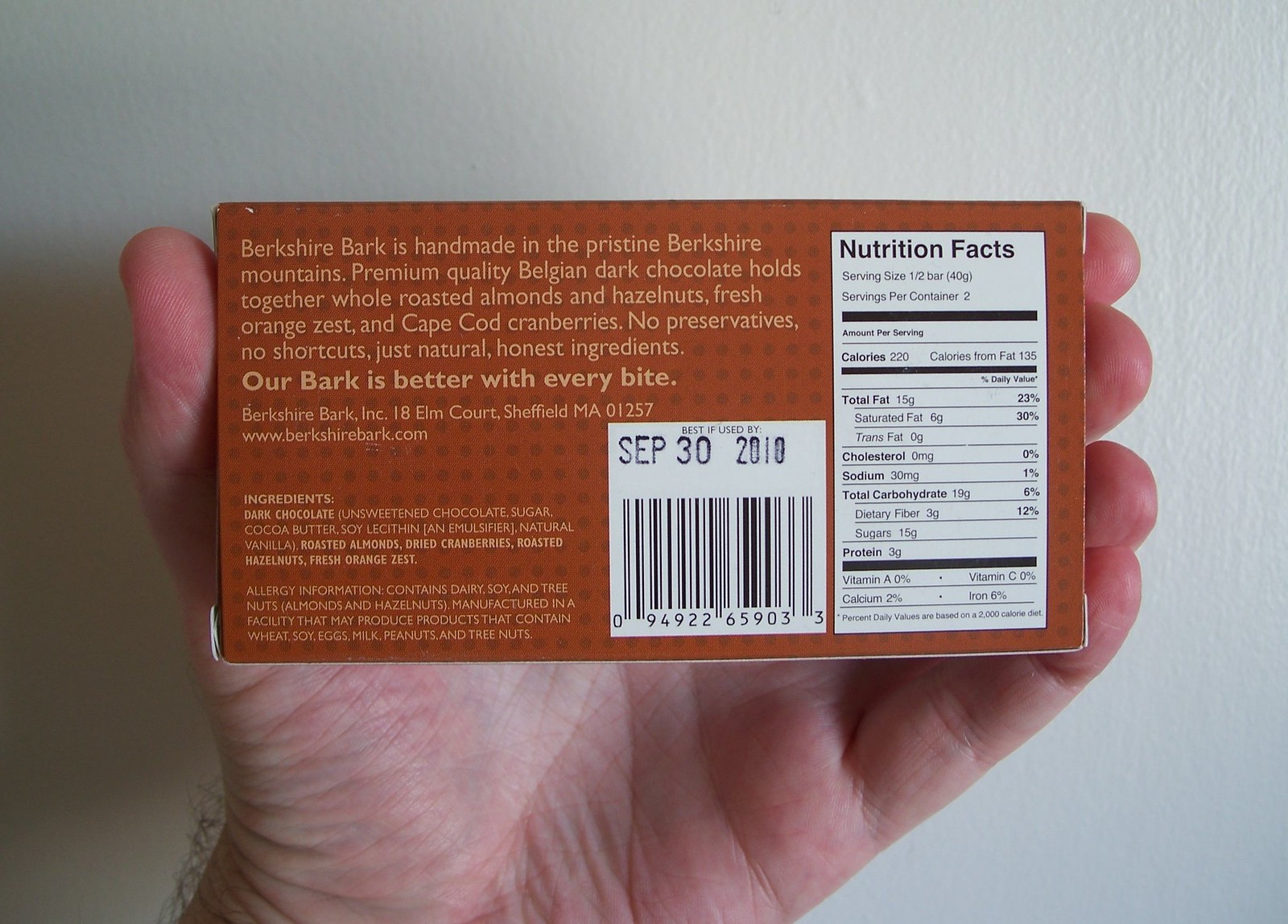This image features a detailed view of a light brown rectangular box of Berkshire Bark dark chocolate being held by a person’s left hand against a grey background. The hand is visible with the thumb and fingers wrapped around the small cardboard box. The photograph shows the back of the box, where several elements are clearly visible. In the upper-left section, there is a paragraph that reads: "Berkshire Bark is handmade in the pristine Berkshire Mountains. Premium quality Belgian dark chocolate holds together whole roasted almonds and hazelnuts, fresh orange zest, and Cape Cod cranberries. No preservatives, no shortcuts, just natural, honest ingredients. Our bark is better with every bite." To the right of this text is a white rectangular area containing the nutrition facts, which include serving information and calorie count. Below this, in the middle, there is a barcode with a stamped date of September 30, 2010. The lower-left corner of the box contains the list of ingredients.